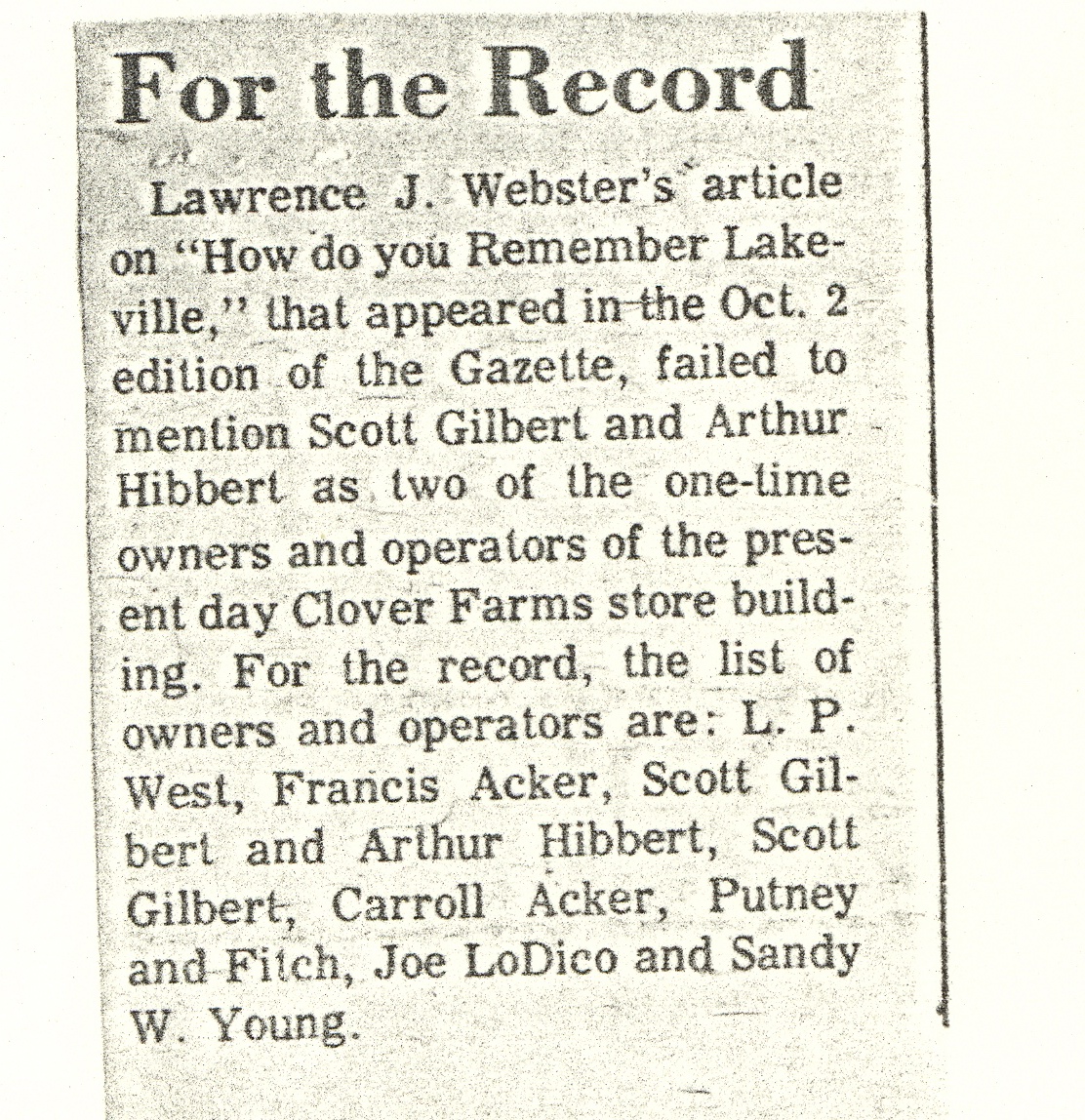The image depicts a faded, black and white clipping from an old newspaper article. The article has an off-white background with black ink text. At the top, in bold black letters, it reads "For the Record." Beneath this heading, the text details that Lawrence J. Webster's article titled "How Do You Remember Lakeville," which appeared in the October 2 edition of the Gazette, failed to mention Scott Gilbert and Arthur Hibbert as two of the former owners and operators of the present-day Clover Farms store building. The corrected list of owners and operators includes L.P. West, Francis (or Carol) Acker, Scott Gilbert, Arthur Hibbert, Putney & Fitch, Joe Lodico, and Sandy W. Young.